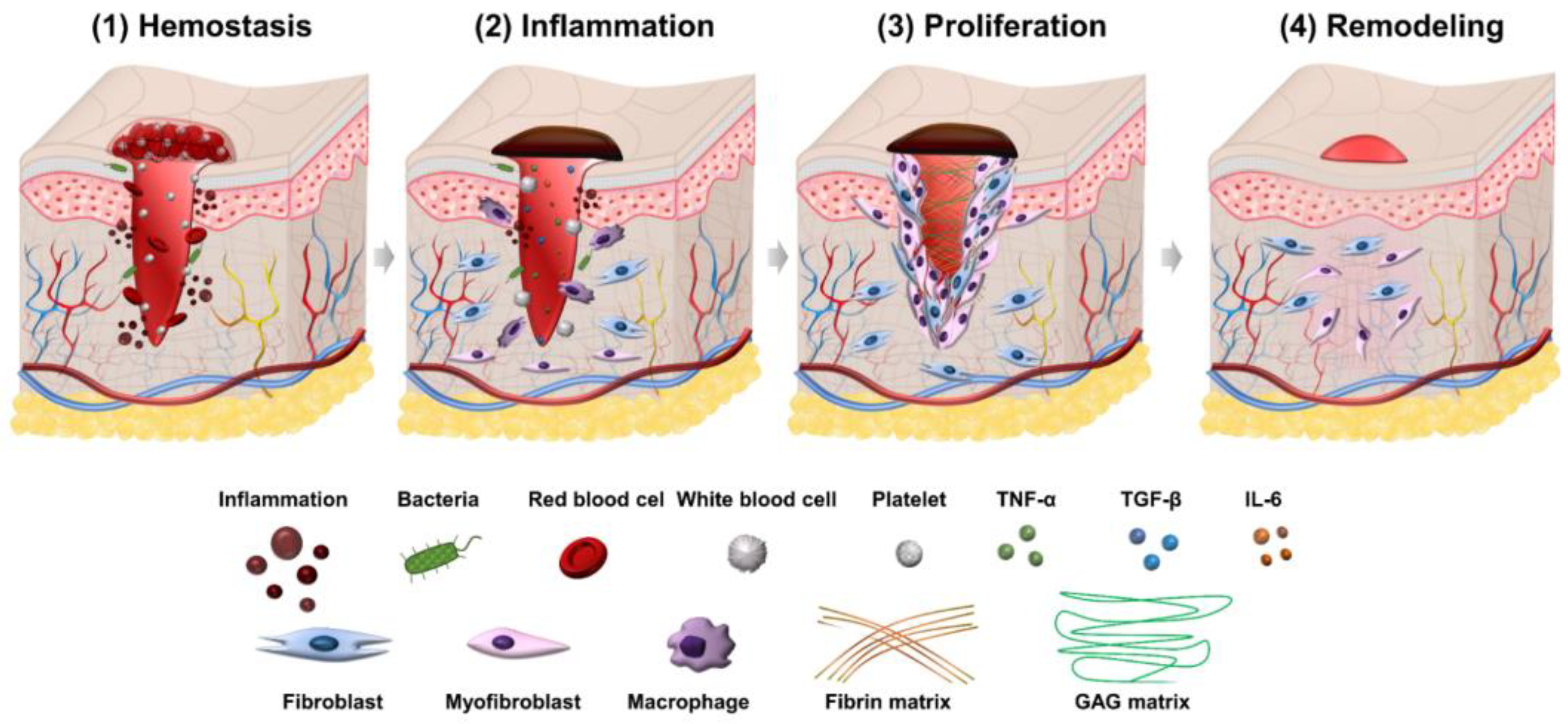The image appears to be an excerpt from a health textbook detailing the stages of a pimple or infection at the cellular level. It features four sections, each showing a cube illustration that visually represents a stage in the disease or healing process: hemostasis, inflammation, proliferation, and remodeling. Each stage showcases a red vertical line, likely representing the infection or injury, extending into what seems to be skin tissue. 

- **Hemostasis**: This stage shows initial inflammation with a red column penetrating the skin, and numerous tiny details resembling blood vessels and cells.
- **Inflammation**: The red column now has a dark brown top, denoting inflammation, and various immune cells like white blood cells and bacteria can be seen around it.
- **Proliferation**: Here, the red column is still present with a brown inflamed top, surrounded by proliferating cells and additional details indicating cellular activity.
- **Remodeling**: The final stage where the red column has disappeared, and the surrounding cells are dispersing, signifying healing or remodeling of the tissue.

The bottom of the image provides labels and illustrations for various cells and molecules involved in these processes, including bacteria, red blood cells, white blood cells, platelets, fibroblasts, myofibroblasts, macrophages, fibrin matrix, GAG matrix, and signaling molecules such as TNF-A, TGF-B, and IL-6.